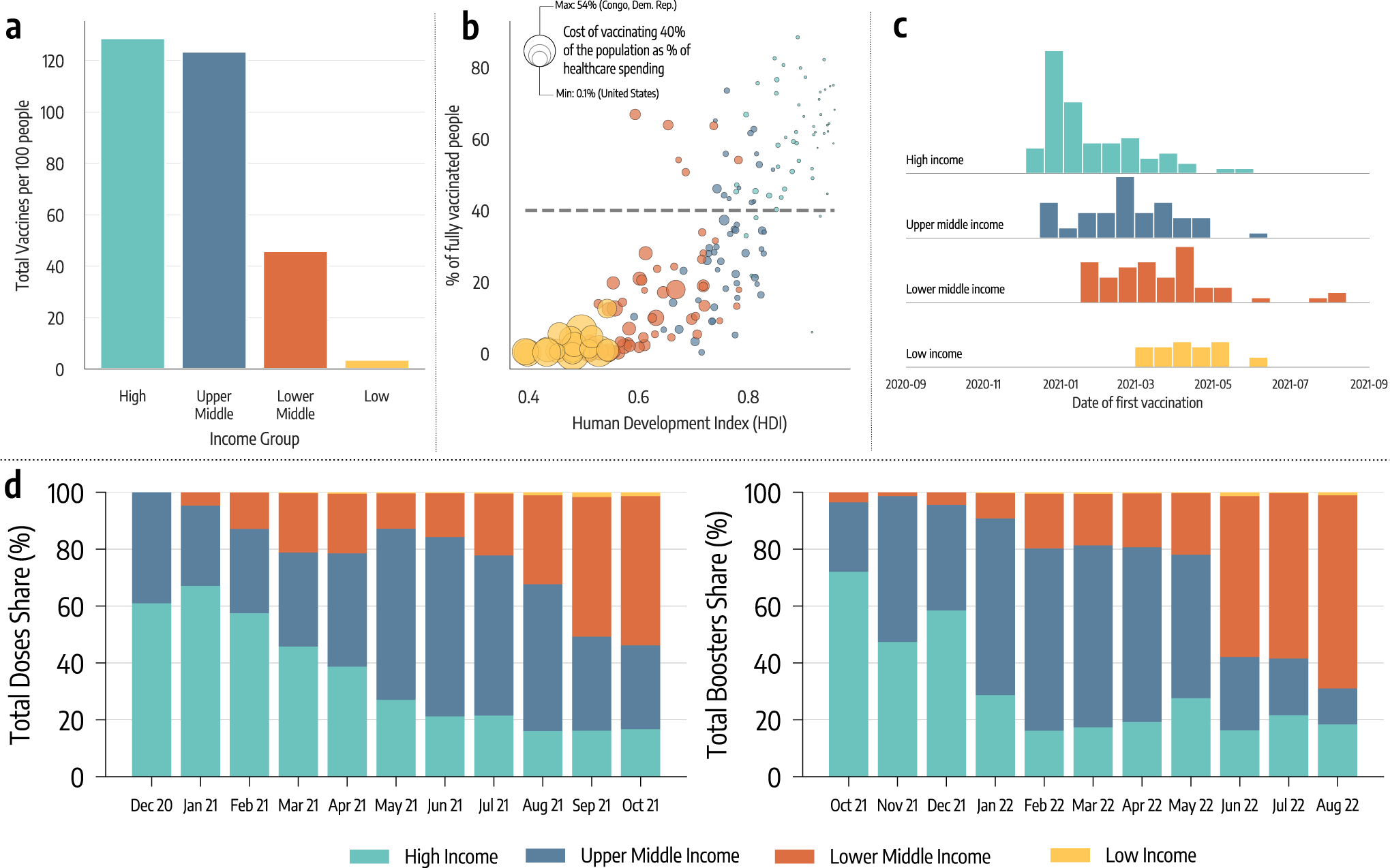The image depicts five detailed charts, each focusing on various aspects related to COVID-19 vaccinations across different income groups and development indices. The first chart on the left visualizes 'Total Vaccinations per 100 People' with bars representing high, upper middle, lower middle, and low income groups, showing a decrease in vaccination rates as income levels drop. The second chart correlates the 'Human Development Index (HDI)' with the 'Percentage of Fully Vaccinated People', suggesting a positive relationship between higher HDI scores and vaccination rates. A third chart details the 'Cost of Vaccinating 40% of the Population as a Percentage of Healthcare Spending' across different income groups. The fourth chart represents the 'Date of First Vaccination', with timelines for high, upper middle, lower middle, and low income groups, indicating that higher income groups began vaccination earlier. The fifth chart displays 'Total Doses Shared Percentage' and 'Total Boosters Shared Percentage' over time, from December 2020 to October 2021, across the same income classifications, highlighting disparities in vaccine distribution and booster administration among the various income levels. Together, these charts offer a comprehensive look into the vaccination inequities influenced by income and development metrics.